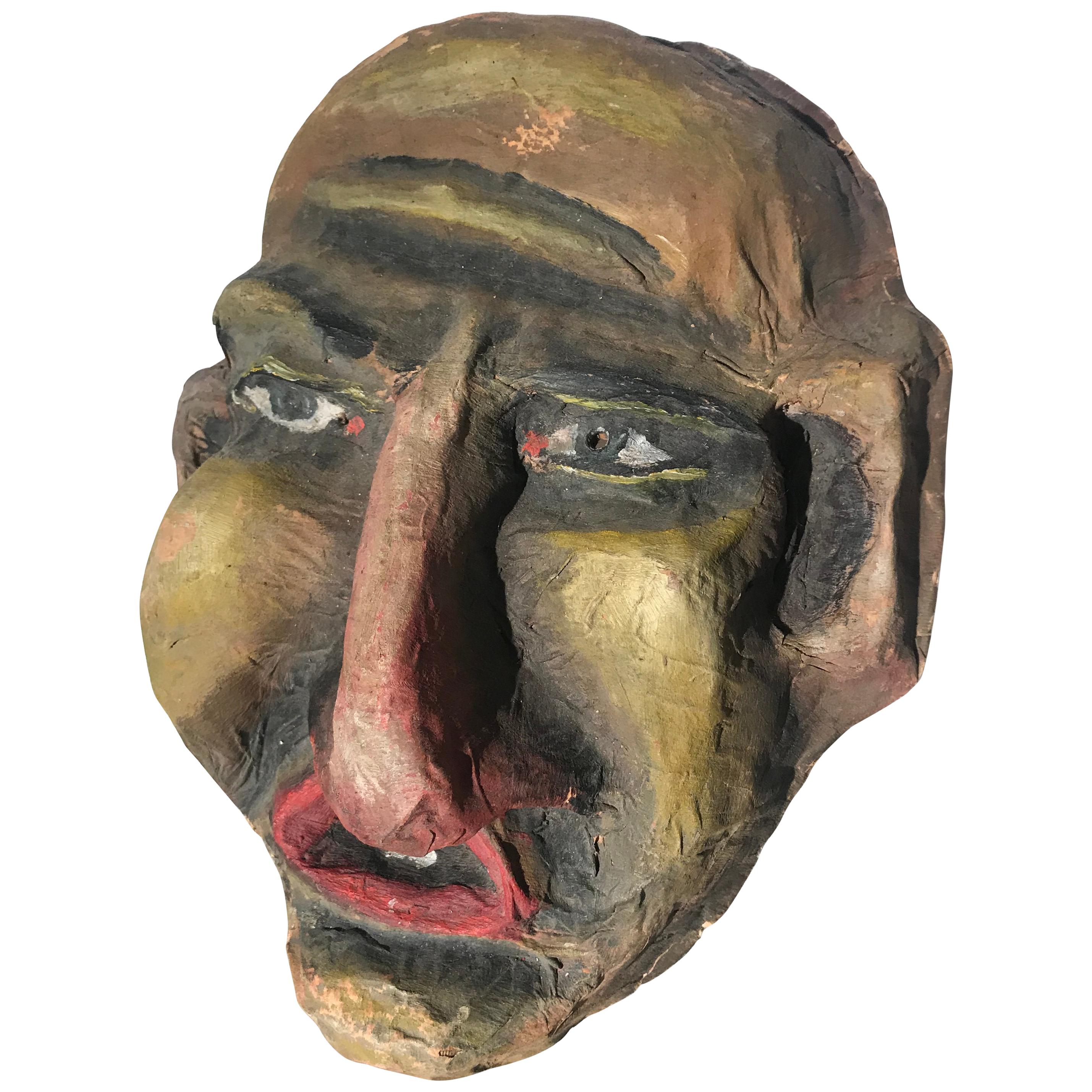This image features a large, homemade mask, likely crafted from clay or paper mache, displaying an intriguing blend of colors and a matte, papery texture. The mask is sculpted into the shape of a human face, characterized by a long brown nose and round, yellow cheeks. The open mouth is highlighted with striking red lips, revealing two small white teeth against a dark interior. The strong, pointy chin and square brown ears frame the face, while the black, jutting eyebrows sit above expressive white eyes with black pupils, accentuated by black makeup. The mask's expressive features include an angular jawline and a rounded forehead. Adding to its vivid appearance, black and green shades cover the forehead, ears, and various other parts of the face, giving it an air of eerie artistry, reminiscent of a Halloween or artistic mask.